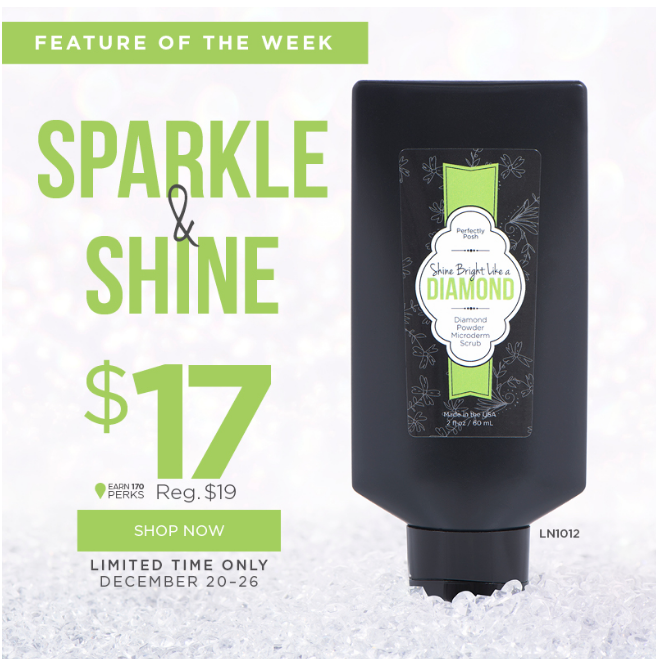This advertisement features a microderm scrub product with a clean white background. At the very top, there's a light pastel green bar with white text reading, "Feature of the Week." Below it, in large bold green letters, it says, "Sparkle and Shine $17," with a small black ampersand. In black letters, it mentions, "Earn 170 Perks Regular $19," followed by a green bar with white text stating, "Shop Now." Beneath that, in black text, there is a note specifying, "Limited Time Only, December 20th through 26th."

On the bottom of the image, there's a crystal-like pattern that resembles diamonds or glass, aligning with the theme of the product. To the right of the image stands an upside-down black squishable bottle. The bottle has a black sticker adorned with white-outlined flowers. Cutting through the middle of the sticker is a green line, featuring a white cloud emblem with the text, "Shine Bright Like a Diamond," where "diamond" is in green and the rest of the words are in black. Beneath this, it says, "Diamond Powder Microderm Scrub."